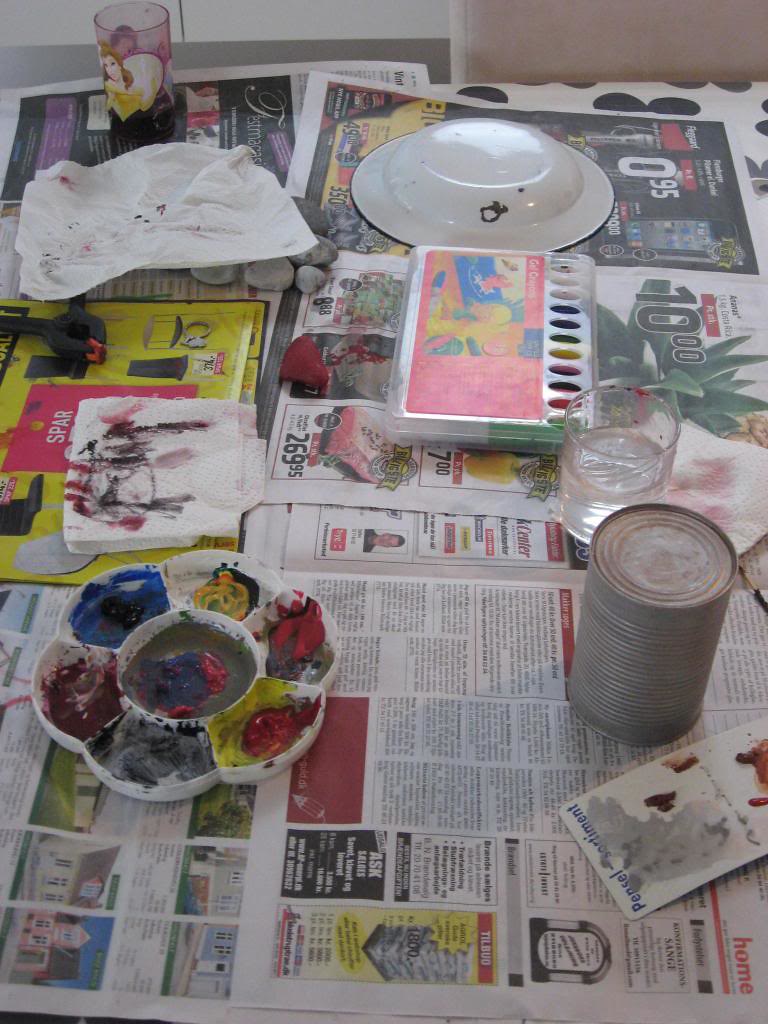This photograph showcases a well-organized painting area filled with various art supplies, set against the backdrop of a table covered with newspaper to protect the surface. The table, white with black polka dots, holds the central focus of the scene: an empty circular tray surrounded by six small cups arranged like petals on a flower. Each cup contains a different color of paint, ready for use.

Among the painting supplies, there is a stainless steel cylinder can, seemingly unopened, resembling a can of spinach without its label. Nearby, an unopened package of pencils and other drawing accessories lie in anticipation of future use. A glass of water, likely for rinsing paintbrushes, and a well-maintained paint set are also present, indicating a committed and tidy artist at work.

Scattered around are a couple of paper towels stained with red and black paint, evidence of brushes being cleaned. In the corner, there is a whimsical princess-themed cup, possibly filled with a beverage like Coke for the artist. Adding a touch of practical makeshift organization, a bowl is positioned upside down, revealing its white underside. The scene vividly captures the essence of an artist's workspace, rich with the tools and colors of their trade.